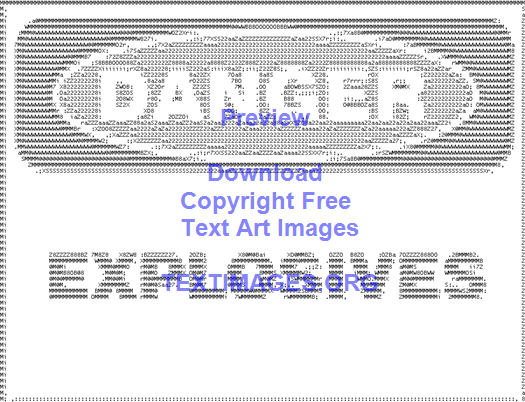This image is a small, rectangular, horizontal danger label available for download. The label features a distinct design with a rounded black rectangle and a lighter interior. At the very top, inside a white oval ring, large white text reads "DANGER." Beneath this, in the white area, large black letters spell out "EXPLOSIVES." Overlaying this foundational text art, semi-transparent blue text states "Preview," followed by "Download," "Copyright-Free," "Text Art Images," and finally, "TEXTIMAGES.ORG," which is slightly harder to read as it is superimposed directly over "Explosives." The entire image is black-and-white text art, and each pixel is represented by characters, creating a unique, detailed depiction.